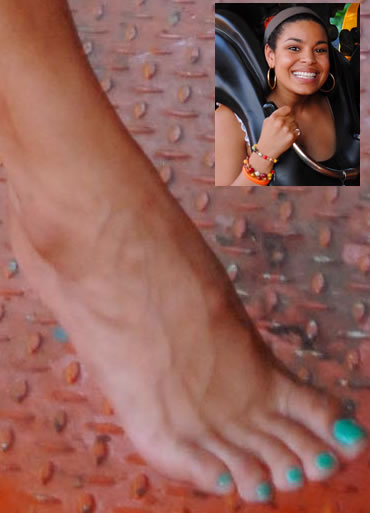The photograph depicts a composite image that captures two distinct sections. In the foreground, there is a close-up of a woman's right foot with light brown skin, poised on a red, textured metal floor exhibiting a diamond plate pattern. Her toenails are painted a vibrant turquoise or mint green color. This foot scene dominates the left side of the image and highlights wear spots on the floor where the original gray metal shows through.

In the upper right-hand corner, there is a smaller, passport-sized photo of singer Jordan Sparks, likely taken from a screen during a FaceTime call or similar event. She is sitting on a roller coaster, secured with large black over-the-shoulder straps. Jordan is smiling broadly at the camera, exuding a joyful vibe. She wears a gray bandana around her head, large gold hoop earrings, and several chunky, beaded bracelets adorn her right wrist, which holds onto the roller coaster rail. Her dark hair is pulled back, emphasizing her cheerful expression as she enjoys the amusement park ride.